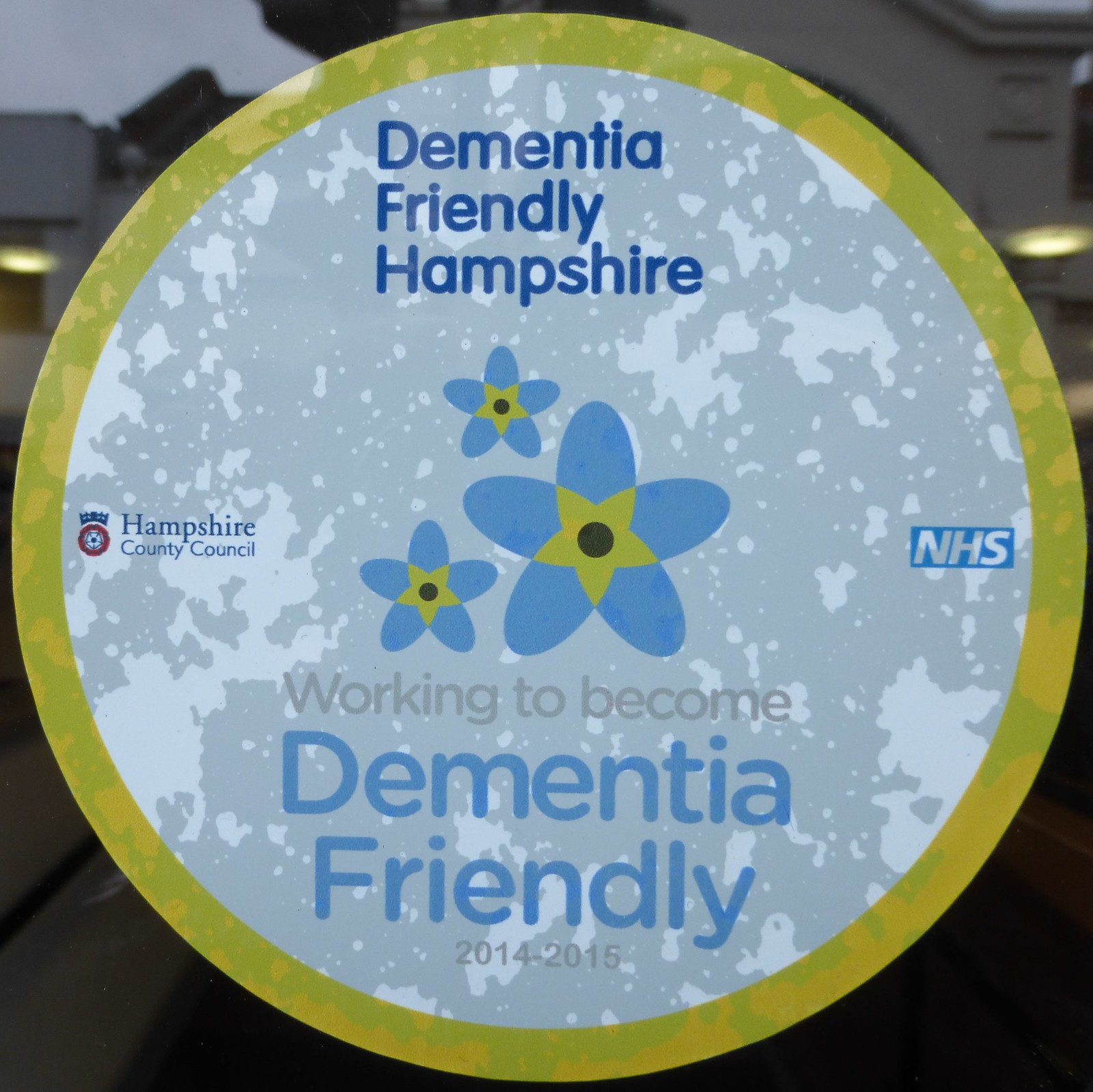This image captures a circular window sticker with a yellow border against a white background, marred slightly by air bubbles. Dominating the upper part of the sticker, in blue text, are the words "Dementia Friendly Hampshire." Centrally positioned are three blue five-petaled flowers of various sizes, each with a yellow center. Below the flowers, gray text reads, "Working to Become," followed by "Dementia Friendly" in blue, and the years "2014 to 2015" in gray. On the left side of the sticker is a small Hampshire County Council logo, with a soccer ball graphic. To the right, against a blue background, the white letters "NHS" are prominently displayed. In the background, some parts of a house or a building can be vaguely discerned through the glass, out of focus.